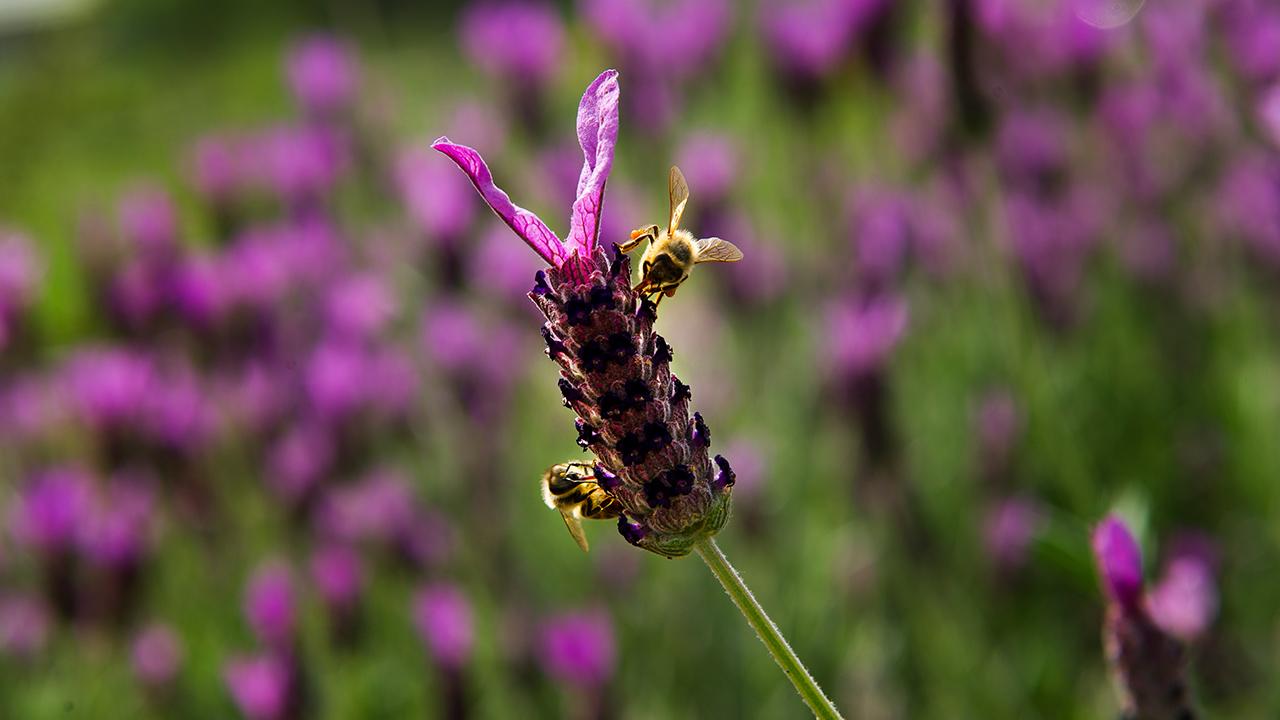This image captures an up-close view of a vibrant purple flower with two bees prominently featured, one on the lower left and one on the upper right, likely engaged in pollination. The flower itself stands out with its green stem and distinctive head, characterized by dark purple specks and two lively purple petals extending from the top. The bees, possibly bumblebees, display sheer wings, matchstick-like legs, yellow fuzz, and black faces. In the background, a blurry field of similar purple-topped flowers and green grass can be seen, adding depth and context to the scene.